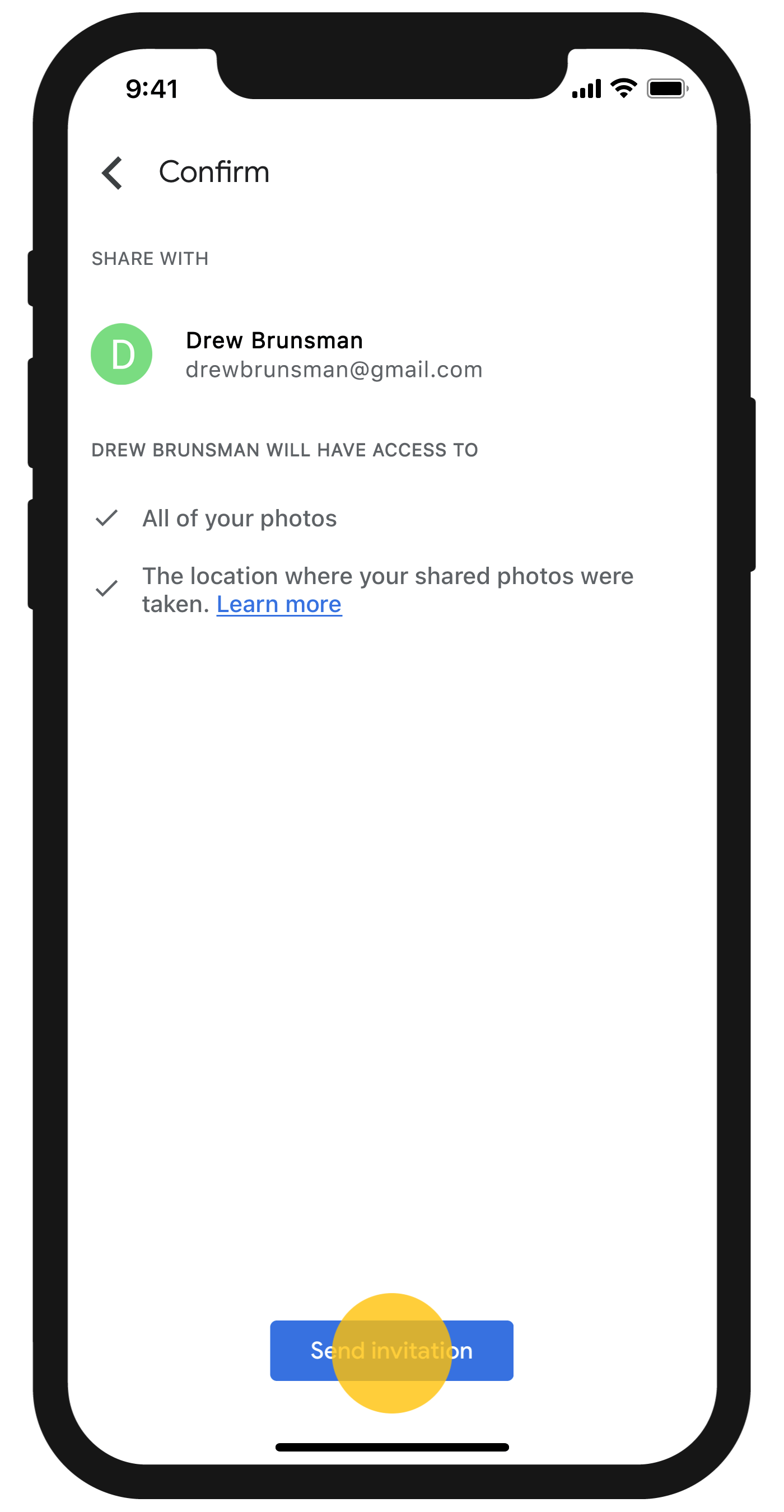The image depicts a close-up of a smartphone screen. The phone has a sleek black border, highlighted by three buttons on its left side: two of the same size and a smaller one positioned at the top. On the right side, a single, elongated button is visible. 

On the screen, the status icons at the top-right corner indicate that the battery is fully charged, and both the Wi-Fi and phone signal strengths are at maximum. The current time displayed at the top-left is 9:41 AM. Below the time, there is a navigation bar showing the word "Confirm" accompanied by a back arrow on its left.

Further down, the phrase "Share with:" precedes the email contact details of Drew Brunsman, displayed as "Drew Brunsman (drewbrunsman@gmail.com)." Adjacent to the email, a green circle icon with a white 'D' inside is visible. 

The text "Drew Brunsman will have access to:" follows, listing two items with checkmarks beside them: "All of your photos" and "The location where your shared photos were taken."

At the very bottom of the screen, a prominent blue rectangular button with the label "Send Invitation" is present, ready to be tapped.